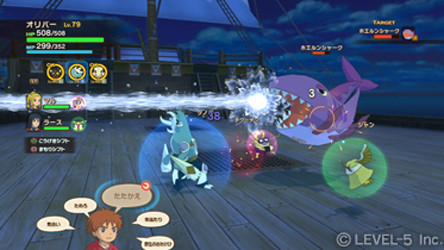This is a screenshot from a computer game with a predominantly blue and purple color scheme. Dominating the center-right of the image is a whale, which is purple on top and blue underneath, with its mouth wide open. Emerging from its mouth is a bright white circular formation, suggesting an orb, which is surrounded by water spraying in a straight horizontal line to the left. Below the whale and to the right, there's a green circle housing a green bell. The bottom floor of the game is colored in shades of gray and blue.

To the left of the whale, there's a blue circle containing a green character with black eyes and a white body. In the lower-left corner, a character with red hair and wearing a red shirt has several word bubbles encircling his head; the bubbles are beige-brown, but their text is unreadable. The background is a mix of bluish-purple hues, likely depicting clouds. Additional details include a black scoreboard with various bars and icons situated in the upper left corner. The scene appears to unfold on or near a wooden dock.